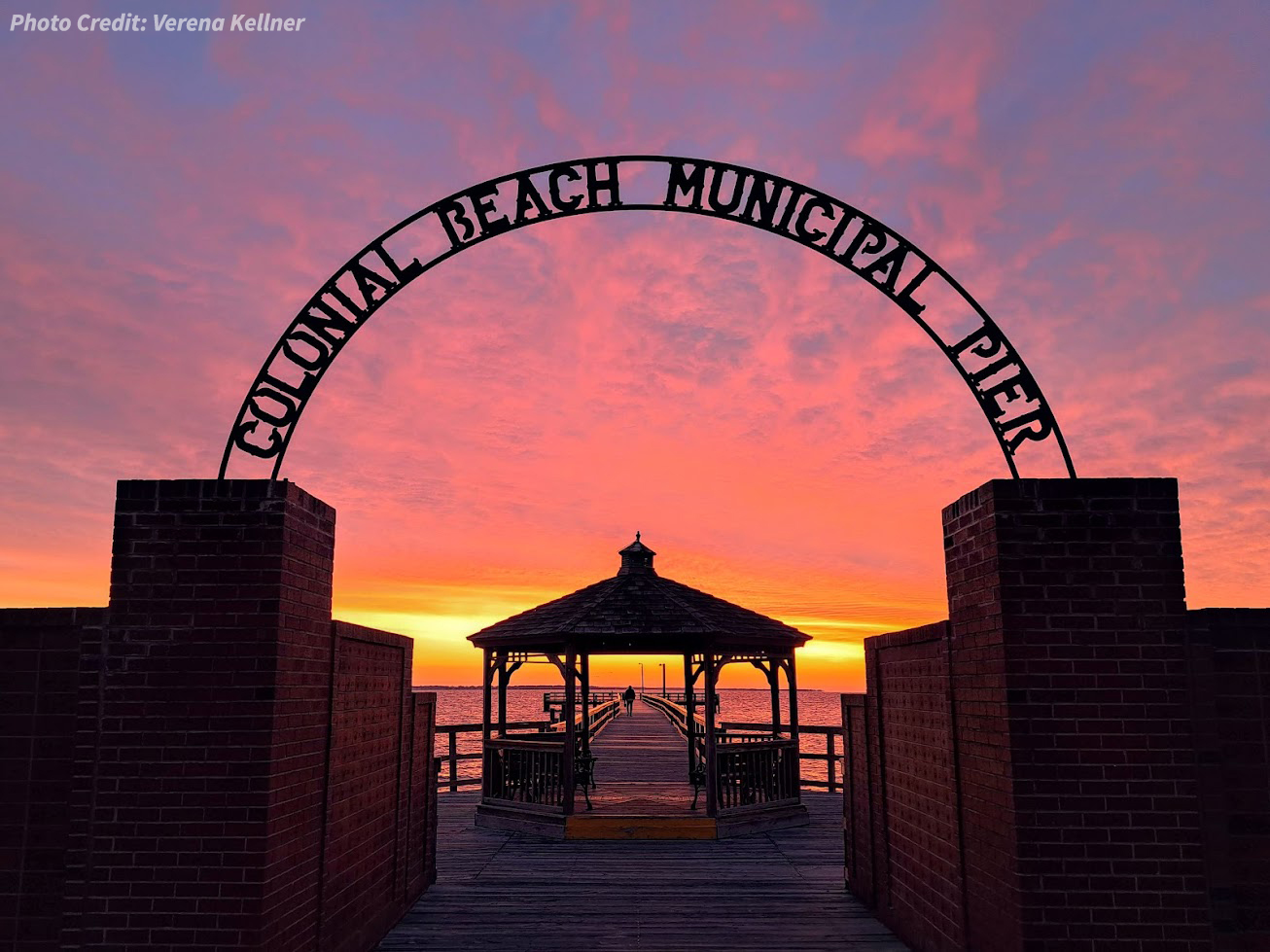The image depicts a breathtaking sunset or sunrise over the Colonial Beach Municipal Pier in California, casting a vibrant array of blues, oranges, yellows, peaches, pinks, and light lavender hues across the sky. The camera captures the scene from the entrance of the pier, showcasing a metal arch rising from two brick columns that frame the entranceway. The arch is inscribed with the name "Colonial Beach Municipal Pier." At the center of the composition is a gazebo, serving as a picturesque gateway that leads the viewer's eye directly through its entranceways to the long boardwalk extending into the ocean. The boardwalk, illuminated by the warm, orange glow of the setting or rising sun, eventually leads to a lone figure standing at the far end of the pier, adding a serene and contemplative element to the scene. The entire composition exudes tranquility, making it an ideal spot for moments like weddings, picnics, or simply basking in the beautiful view of the ocean.